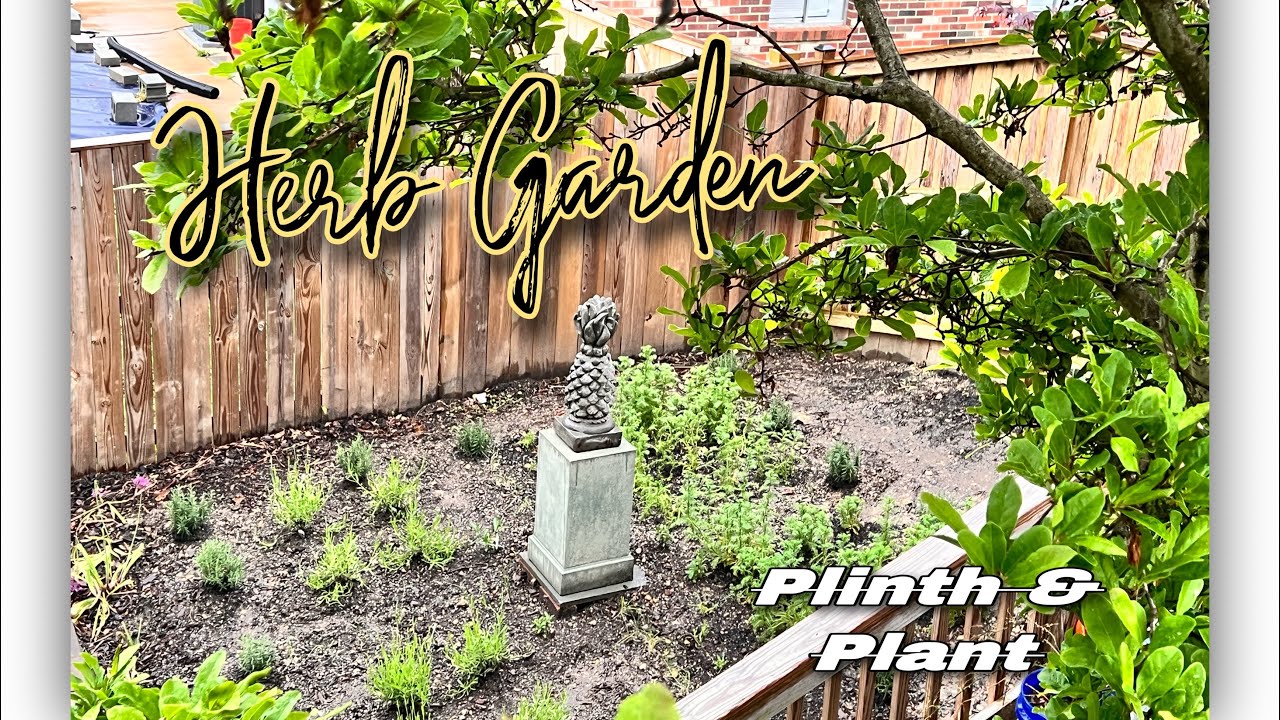The image captures a picturesque herb garden, bordered by a brown wooden picket fence that extends horizontally across the background. The photograph, possibly taken from a slightly elevated position, looks down upon an area of bare earth interspersed with neat rows of small, young herb plants. The plants vary in hue from dark to light green and are arranged systematically throughout the plot. Dominating the scene is a large tree with sprawling green branches that partially shade the garden. In the middle of the garden stands a decorative statue of a pineapple, perched on a stone plinth. Along the top of the image, in large, elegant cursive letters, the words "Herb Garden" are written in black and yellow. In the lower right corner, the name "Plinth and Plant" appears, suggesting this image could be part of an advertisement for the company.